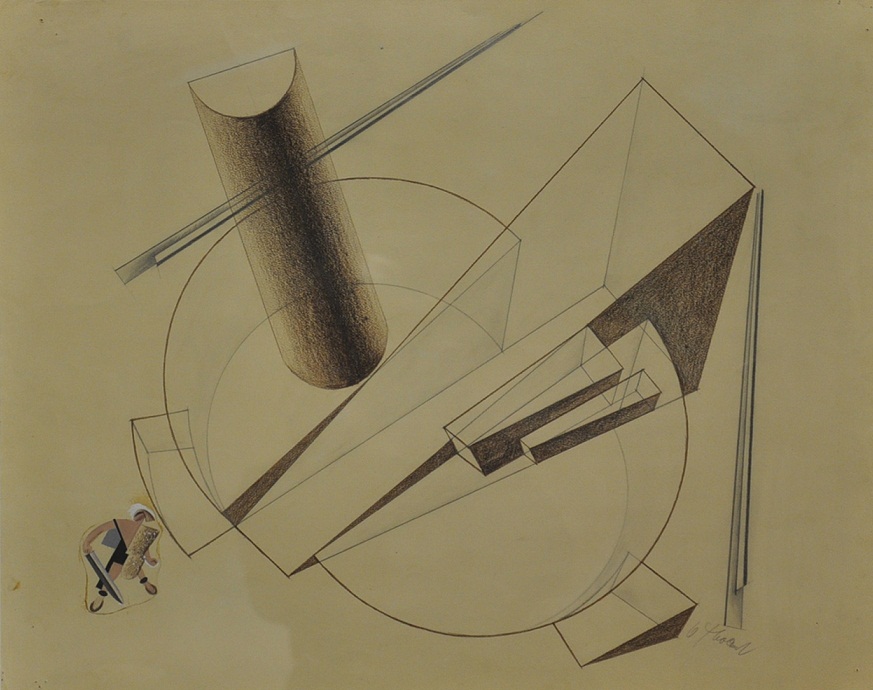This abstract illustration is filled with a variety of geometric shapes including circles, cylinders, triangles, rectangles, and semicircles, rendered primarily in line work with some shaded areas that give volume, particularly to the cylinders. The overall composition emphasizes a geometric style, with a noteworthy focus on the use of lines. A standout is the lower left section, featuring a stylized figure resembling a warrior or hunter, armed with a sword and clad in a loincloth or possible armor, further enhanced by sandals. This figure is depicted in the same abstract and geometric manner and appears to interact with a complex, geometric mass that could be interpreted as a ramp or small colosseum-like structure. The background is subtly shaded in hues of green and gray, and the artist's signature is prominently placed in the bottom right corner. All these elements are meticulously drawn on a piece of paper, contributing to the overall cohesive yet dynamic abstract theme.